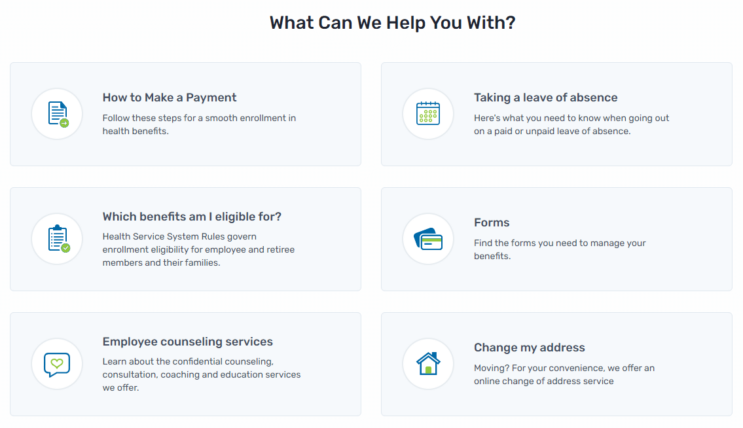The image is a detailed section from a health insurance website, featuring a clean white background and organized layout for user assistance. The design consists of two columns and three rows of light blue, horizontally oriented rectangular text boxes.

At the very top of the image, a prominent, centered header in bold black text reads "What Can We Help You With?" with each word capitalized.

In the first row:
- The left text box, labeled "How to Make a Payment," provides steps for a smooth enrollment in health benefits. It includes a white circle icon with a blue and green document motif.
- The right text box, labeled "Taking a Leave of Absence," offers essential information for employees considering paid or unpaid leave. It is accompanied by a white circle icon featuring a blue and green calendar page.

In the second row:
- The left text box, titled "Which Benefits Am I Eligible For?" is paired with an icon of a clipboard.
- The right text box, titled "Forms," has an icon depicting sheets of paper or cards.

In the third row:
- The left text box, "Employee Counseling Services," includes an icon of a speech bubble with a heart inside it.
- The right text box, "Change My Address," is marked with a home icon.

Each box clearly separates and highlights a specific topic, adorned with easily recognizable icons to aid user navigation.